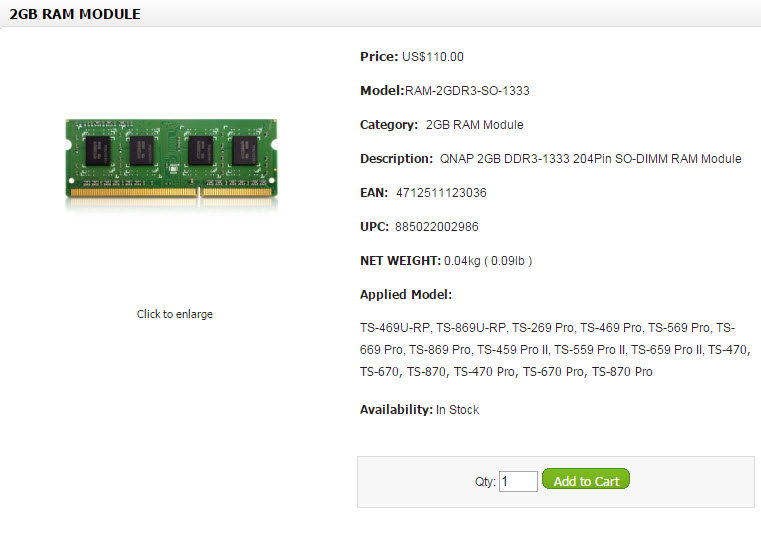**Product Page Screenshot: 2G RAM Module**

The image is a screenshot focusing on a portion of a product page, missing the retailer's header and footer. The top section showcases "2G RAM MODULE" in black, bold, capital letters against a light gray border. The rest of the page features a white background.

In the middle, a detailed list of product specifications is displayed. To the left, an image of the product is visible: a green rectangular RAM module with four black squares evenly spaced across its surface, small white etchings, and a gold border at the bottom.

To the right of the image, the product details are listed as follows:
- **Price:** US $110
- **Model:** RAM-2GDR-SO-1333
- **Category:** 2G RAM Module
- **Description:** Followed by a long string of letters and numbers
- **EAN:** A list of numbers
- **UPC Code:** Another list of numbers
- **Net Weight:** 0.04 kilograms (0.09 pounds)
- **Applied Model:** A long list of letters and numbers
- **Availability:** In stock

At the bottom of the page, a gray rectangle contains a white rectangle displaying the number "1" next to "QTY" for quantity, followed by a green button with rounded edges labeled "Add to Cart."